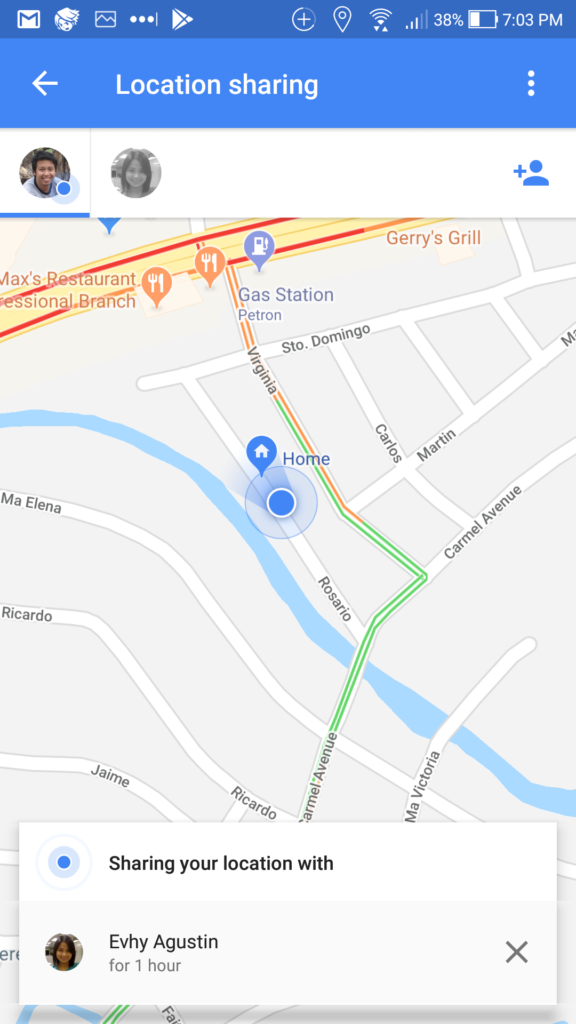A person is using Google Maps to view location details in their local area. The screen shows they are currently sharing their location with another user named Evy Agustin for one hour. Evy's profile picture is that of a young woman, and the person sharing their location, who appears to be around her age, also has a profile picture visible. They both seem to be either high school or college students. On the map, there is a marker indicating the sharer's home address, showing that they are currently at this location. Nearby, there is a marker for a place called Max's Restaurant. The streets in the vicinity feature names like Rosario and Ricardo, suggesting that the area might be in a Latin American country due to the Spanish naming conventions.